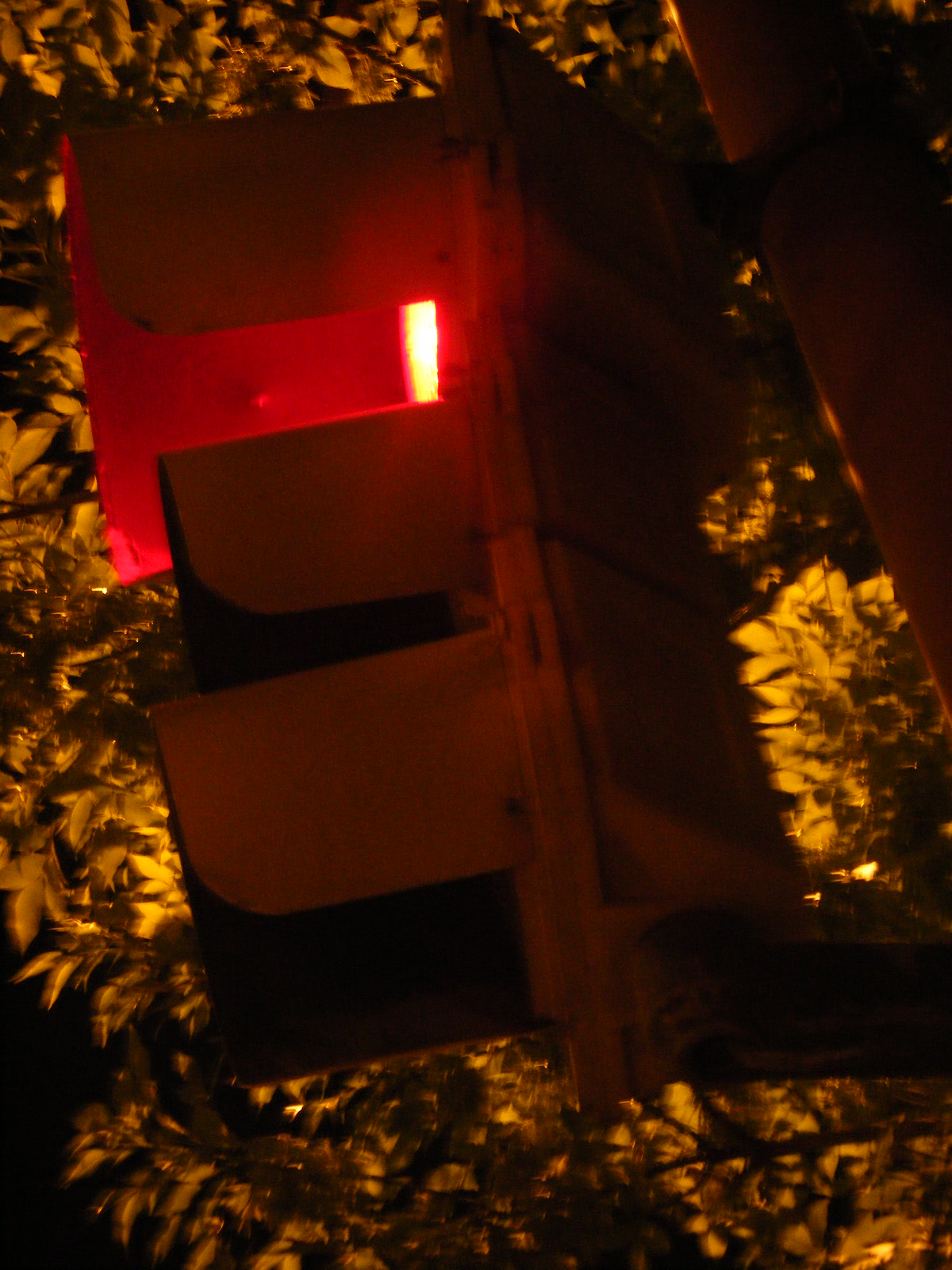This image captures a vivid red structure, likely a birdhouse, adorned with both vertical and horizontal elements, reminiscent of flaps or vents, equally distributed on both sides. The birdhouse is nestled within a tree, which itself is festooned with sparkling lights, enhancing the enchanting ambiance of the scene. Inside the birdhouse, a gentle light illuminates its interior, casting a warm glow through the flaps. A person's arm, visible in the image, suggests that they might be in the process of hanging or adjusting the birdhouse. The structure's vibrant red color stands out against the natural backdrop, and the possibility that it could also serve as an insect-zapping lantern adds to its intriguing functionality.